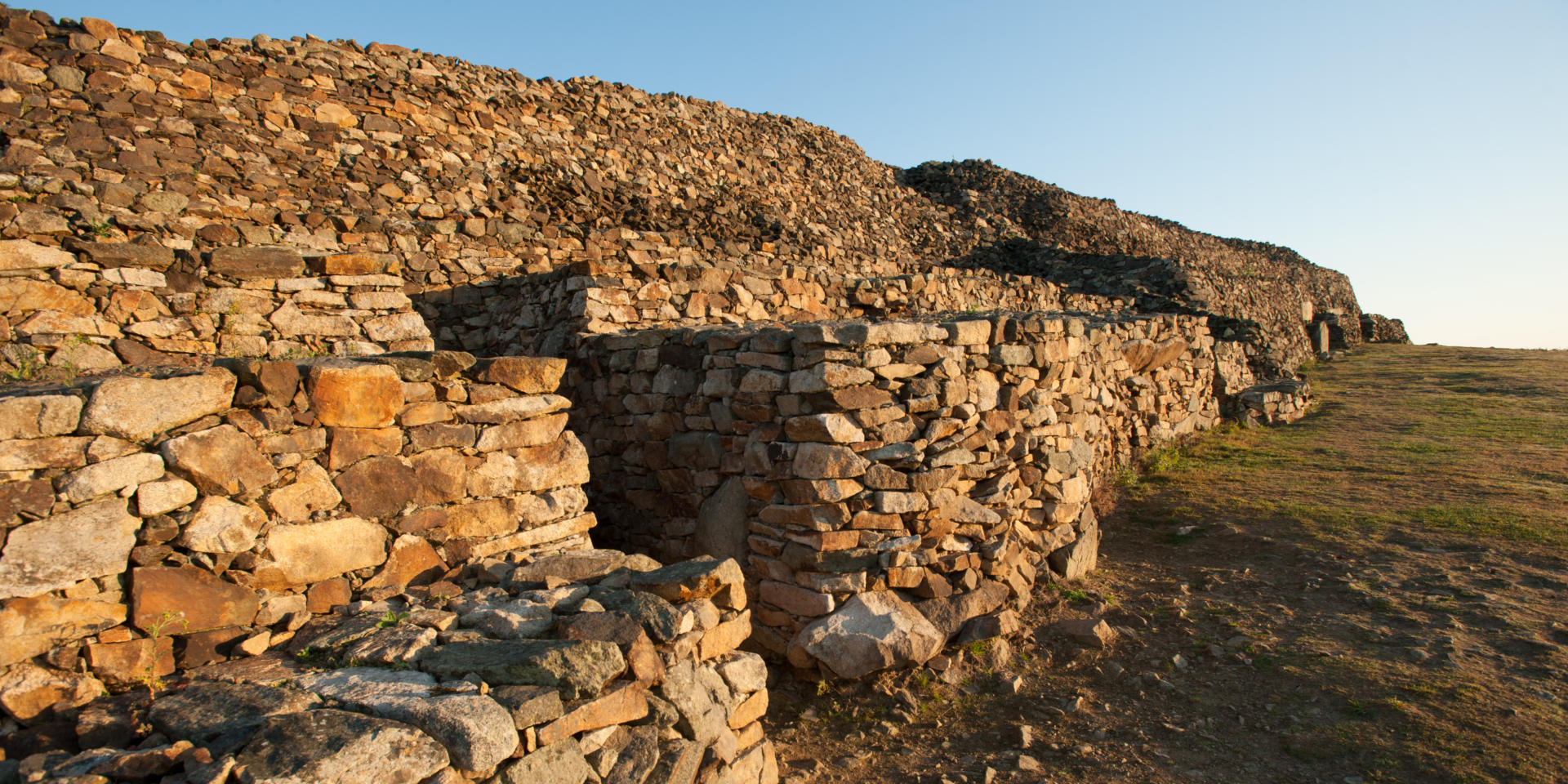This photograph captures a sprawling, primitive ruin of stacked stones and bricks situated in a desolate field. The structure, possibly an ancient fort or root cellar, appears to be in disarray, resembling a large, elongated pile of rocks with traces of organized construction. The central feature stretches diagonally across the image, diminishing from the bottom right to the center left. The stones vary in color, ranging from orangish-gray and brown to lighter gray, with deeper shadows casting some stones in darker hues of gray and black. An entrance can be seen to the left, framed by rocks that fit seamlessly together. The foreground is a dirt surface interspersed with small rocks and patchy grass, gradually leading to the horizon. The sky above is clear and bright blue, suggesting a sunny day without visible clouds. The landscape, though marked by scattered vegetation, further emphasizes the ancient and weathered state of this vast, rocky structure.